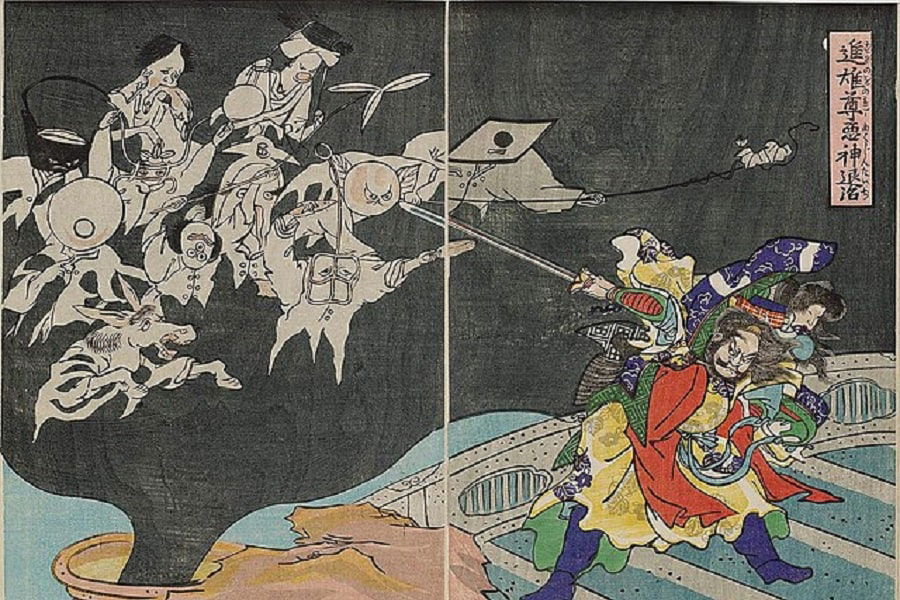The image depicts a vibrant and intricate scene featuring a traditional Chinese warrior engaged in a fierce battle against ghostly demons emerging from a black, smoky haze. The warrior stands prominently in the lower right corner, adorned in a multi-colored robe of red, yellow, green, and blue, with blue boots. His right arm is extended upwards, wielding a sword aimed at the ethereal demons. His facial expression is intense, emphasized by his mustache, long hair, and a distinctive hat that resembles a scarf wrapped around his head in green, red, and blue hues. The setting includes a detailed floor pattern of green and brown panels and a slight concrete-colored wall behind him.

The background, predominantly gray with a black section above the warrior's head, is punctuated by vertical Chinese characters descending from the upper right corner towards the center. These characters suggest a historical ambiance, potentially from the 1500s. Emerging from the black smoke in the lower left corner of the image are various indistinguishable figures, including shapes resembling horses, people, and chariots, contributing to the eerie and chaotic atmosphere.

Despite the predominantly monochromatic background, there is a rich tapestry of colors in the warrior's attire and the ghostly figures' lavender-tinged apparitions. The scene evokes a timeless battle between order and chaos, richly detailed and brimming with historical and cultural references.